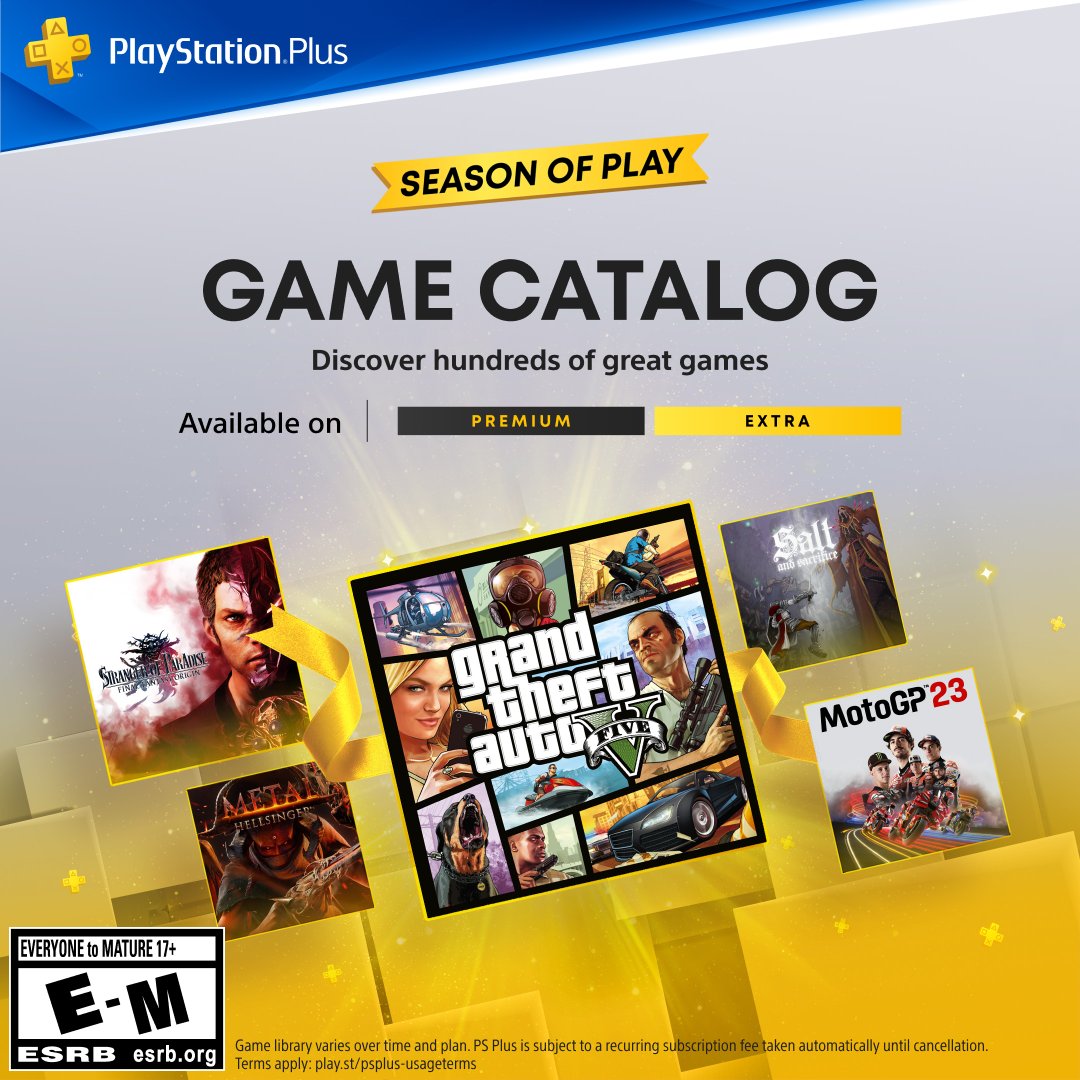In the upper left corner of the image, the background color is blue, featuring a yellow directional pad with four distinct symbols: a triangle, a circle, an X, and a square. Adjacent to this is the PlayStation Plus logo. Below this, there is a gray section with a yellow banner across it, displaying the text "Season of Play." Underneath the banner, in bold black text, it reads "Game Catalog," accompanied by the tagline, "Discover hundreds of great games."

Further down, the phrase "Available On" is presented, followed by two boxes: a black box containing the word "Premium" in yellow, and a yellow box containing the word "Extra" in black. 

The central portion of the image showcases game covers from the PlayStation catalog. Prominently featured in the middle is "Grand Theft Auto V," depicting various characters, including a man holding a gun, a woman adorned with jewelry, and a dog barking. To the left is another game featuring an anime character, and to the right is "MotoGP 23," which displays riders on motorcycles.

In the bottom left corner, ratings information is provided: "Everyone to Mature 17+" (E–M), followed by "ESRB" and the website "ESRB.org" in all capital letters.